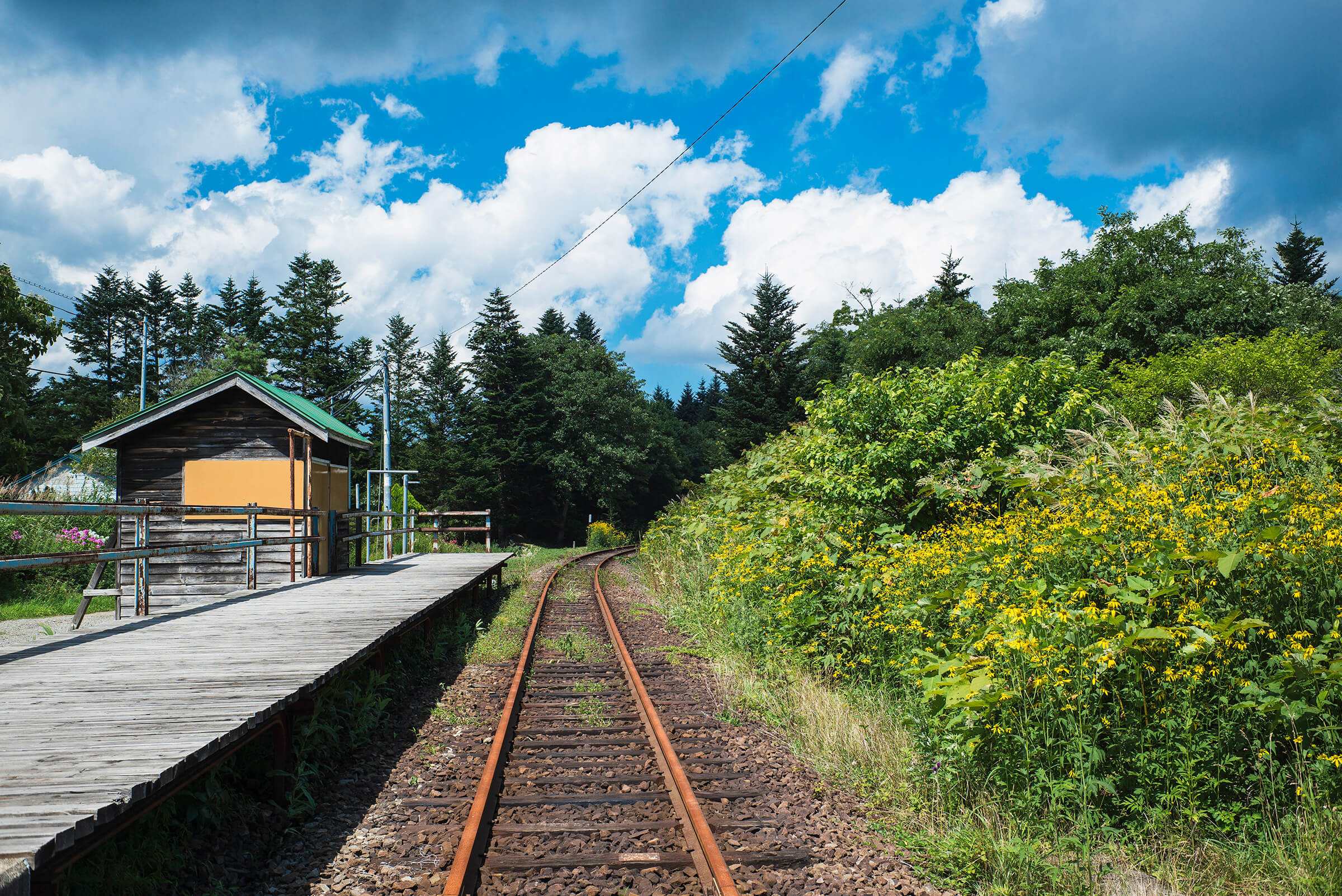In this vibrant outdoor photograph, captured under bright sunshine, an old, rusting railroad track snakes off into the distance, curving slightly to the right. On the right, bushes and yellow flowers abound near the tracks, which bend and disappear around a corner. The tracks themselves are flanked by a charming mix of evergreen pine trees and a scattering of more yellow flowers in the foreground. 

To the left, a small, weathered train station made of gray, aged wood stands on a platform parallel to the tracks. The train station, with its green pitch roof, has a faded yet intriguing appearance, featuring patches of bright yellow panels and a number of pipes and posts emerging from its structure. A rust-coated, formerly blue railing runs in front of the station, and a fence delimits the platform area. The station, presumably used for loading and unloading or perhaps for passenger boarding, includes a small boarded-up house or shack, which might have served as a ticket office or concession stand in the past.

Beneath the tracks, old wooden ties are rotting amidst gravel mixed with brown and white stones, with tufts of grass sprouting through. The landscape is surrounded by an abundance of trees and the sky overhead is predominantly blue, adorned with puffy white clouds. The scene is imbued with a nostalgic charm, capturing a colorful, serene, and beautifully dilapidated piece of history.